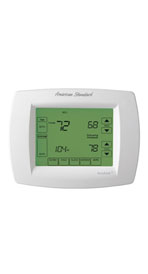In this image, there is a thermostat encased in a white housing with an unreadable script logo. The screen of the thermostat is illuminated with a green backlight and displays various numerical values in black, seven-segment characters. Prominently, the large digits at the upper left read "72," and at the upper right, "68." The bottom left of the display shows "104," and the bottom right reads "78." Adjacent to the "68" on the upper right are black up and down arrows for adjusting the temperature setting. Similarly, up and down arrows are present near the "78" at the bottom right. The display likely indicates the current temperature and separate setpoints for heating and air conditioning, possibly corresponding to different modes such as daytime and nighttime settings. The value "104" appears excessively high, indicating it might be an error or a setting that needs adjustment.